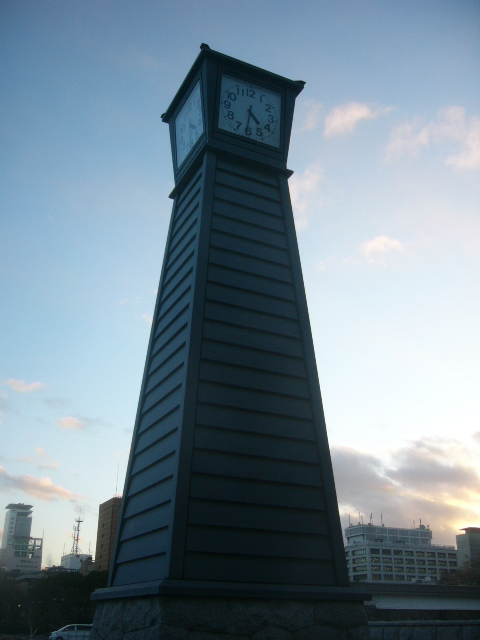This is a detailed colour photograph taken outdoors, capturing an impressive clock tower. The main structure of the tower is made of wooden planks laid horizontally and has a slightly trapezoidal shape, being wider at the base and tapering slightly as it ascends. Standing approximately 5 or 6 meters tall, the clock tower's segmented design gives it the appearance of a tall rectangular prism with indented grooves rising upward. At the tower's summit, a cube-shaped clock, slightly wider at its top due to outward-fanning sides with decorative edges, displays four faces, each marked by conventional numbers from 1 to 12 and black hands on a white background. Currently, the clock shows the time at half past four.

The perspective of the photograph looks up towards the top of the tower, emphasizing its height and providing a striking view of the sky above. The sky transitions from a darker blue at the top to a lighter shade near the horizon, with a section on the right that is overexposed and almost completely white. There are scattered clouds, heavier in the lower right corner, underlit by a subtle yellow glow from the setting sun.

In the background, at the lower edges of the image, a bustling cityscape is visible with modern office blocks, hinting at a city centre business district. Further details include a distant body of water, possibly a river or lake, and a car positioned in the lower left portion of the photograph. This clock tower appears to be a prominent feature, perhaps in a busy city centre or a well-known tourist destination.